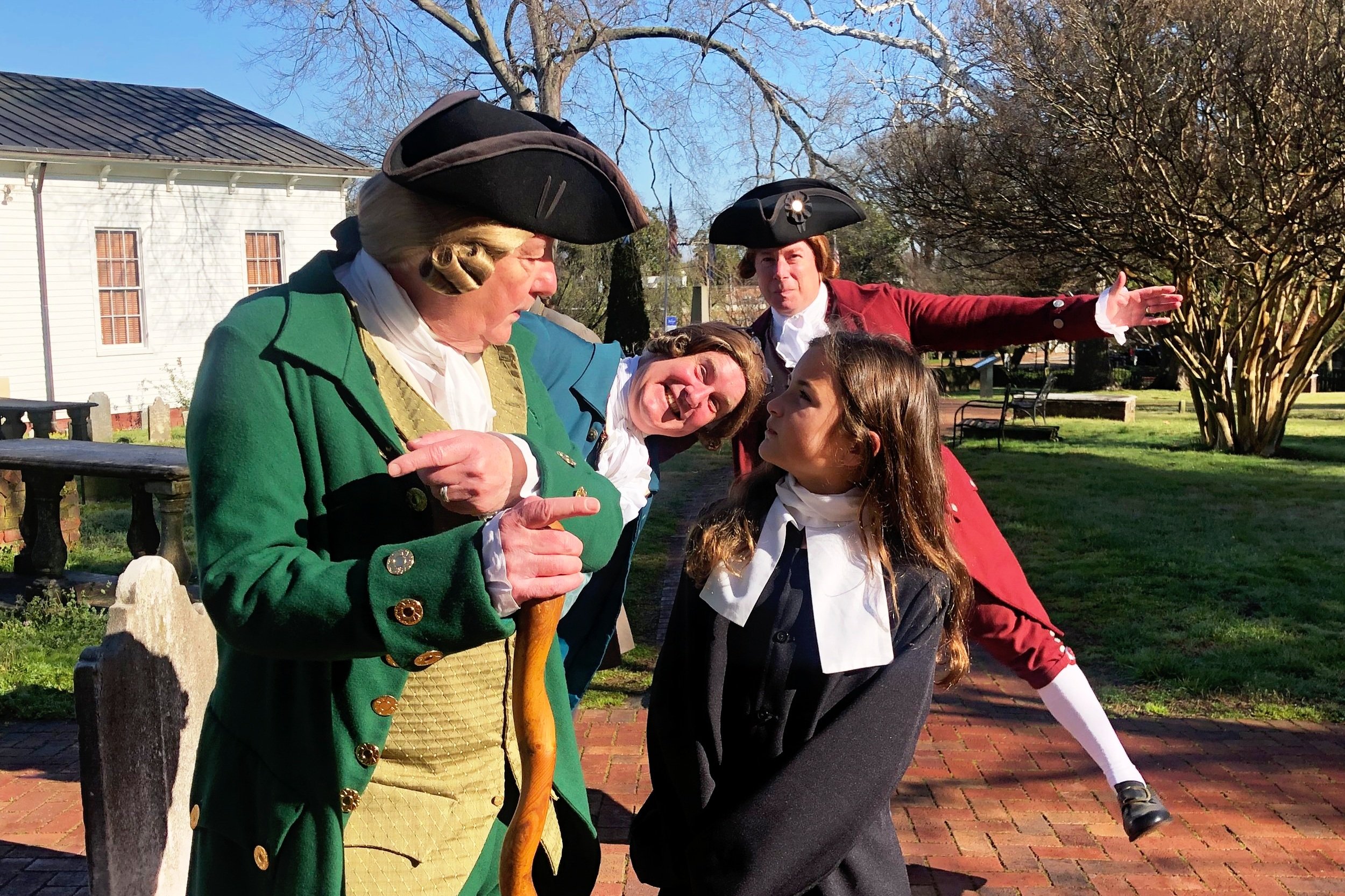In this lively outdoor scene, a young girl with long brown hair, dressed in a dark blue overcoat and a white scarf, stands on a red brick pathway. She’s surrounded by three middle-aged white men, all in vibrant 18th-century, Revolutionary period attire. The men wear wigs and tri-corner hats, and each sports a distinctive color: one in a bright green overcoat with golden buttons, another in a blue jacket, and the third in a red jacket and matching red pants, accessorized with white tights. They stand in silly, animated poses, while the girl, with a bored expression of disbelief, looks up at the man speaking to her. The background reveals a lush green lawn, a cluster of trees mostly bare of leaves, and a traditional white wood-frame building featuring large rectangular windows, white trim, and a black roof. The playful interaction contrasts with the historical setting surrounding them.